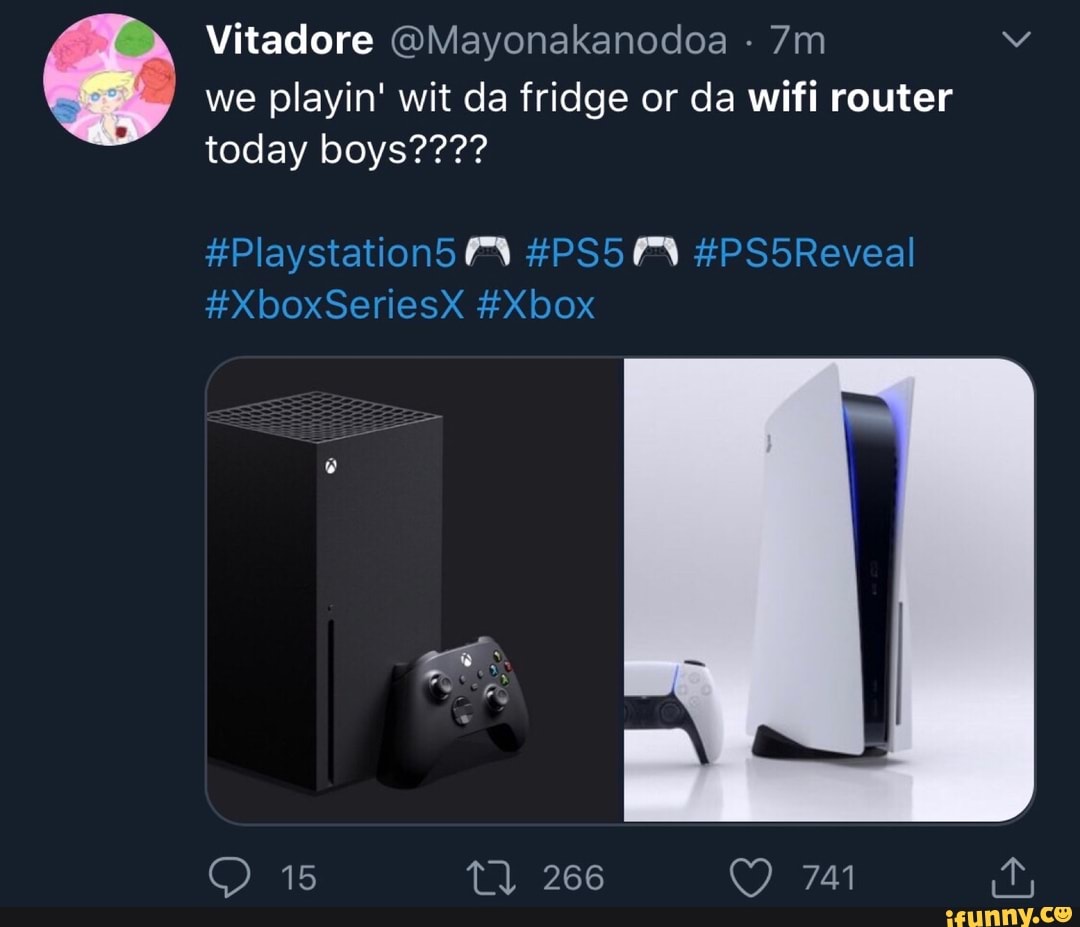In the image, there is a black, tall rectangular PlayStation 5 console with a matching black controller on the left side, and a white, slim, tall rectangular Xbox Series X console with a matching white controller on the right side. The caption humorously compares the sleek designs of the new gaming consoles to household items like a fridge or a Wi-Fi router, reflecting the playful anticipation of deciding which console to play with today. The social media post includes hashtags like #PS5, #PS5Reveal, #XboxSeriesX, and #Xbox to engage the gaming community. The image has garnered considerable attention with 15 comments, 266 shares, 741 likes, and an upload symbol indicating its popularity and reach.